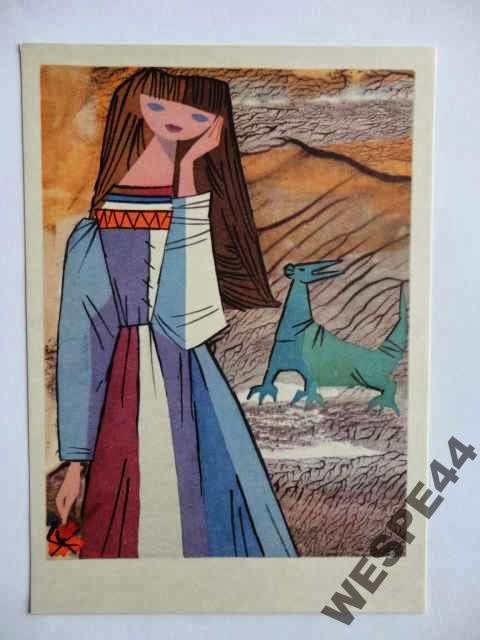This artwork features a cartoonish depiction of a young girl with long brown hair flowing down to her waist, set against a light brown and gray background that resembles rocks. The piece, which is attached to a white piece of paper, includes various intricate details. The girl stands in a field, dressed in a striped, multi-colored dress with long sleeves. The top part of her dress is adorned with purple and white stripes, while the skirt features maroon, white, and various shades of blue and purple stripes. Her left hand rests against her cheek, accentuating her small blue eyes and the subtly distorted triangle-shaped head and neck.

Next to the girl, an abstract aqua-colored creature, possibly a dragon or dog, adds an air of mystery and whimsy to the scene. The creature's darker blue front contrasts with its lighter green back, and it stands with its pointed head directing to the side. The entire image is framed in light gray and blue, contributing to its cohesive presentation. Text in the lower right corner of the artwork reads "WeSPE44" in black.